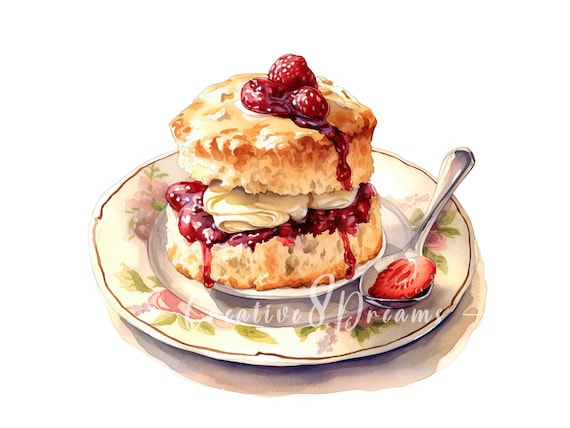This image depicts a detailed watercolor painting of a piece of strawberry shortcake elegantly arranged on a pink floral plate. The plate, rimmed with a golden circular line around the edge and a white center, carries the inscription "Creative Dreams" across the bottom. The shortcake appears to consist of two golden-brown biscuit halves, with a generous filling of strawberries and cream nestled in between. The top biscuit is adorned with additional strawberries and rivulets of strawberry juice cascading down its sides. Beside the shortcake, a silver spoon rests on the plate, holding a single slice of strawberry. The entire presentation exudes a delicate and dreamy aesthetic, characteristic of an artist's rendering.